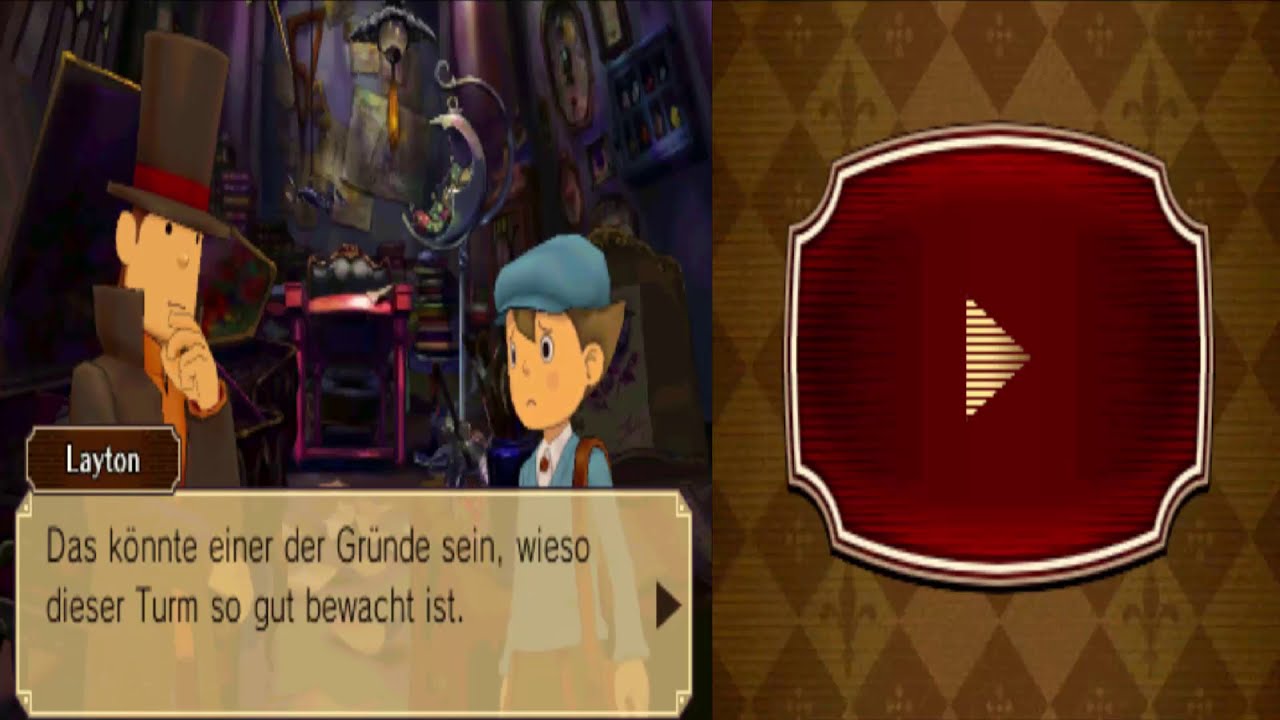The image is divided into two halves. On the left side, there is a detailed screenshot from a video game cutscene. It features two cartoonish characters. The character on the left is a tall, light-skinned man wearing a dark brown top hat with a red stripe and a matching high-collared jacket. He has a confused expression, with his left hand thoughtfully placed on his chin, and he is looking towards the top center of the scene. Beside him is a shorter, younger boy dressed in a blue cap, a blue vest, and a white undershirt, with a brown leather satchel slung over his shoulder. The boy has a worried expression and is also looking towards the center of the image. The setting appears to be a cluttered interior with a crescent moon-shaped statue and various items like books scattered around, giving it a junkyard-like atmosphere. German text bubbles are visible at the bottom, reading: "Leighton das könnte einer der Gründe sein, warum dieser Turm so gut bewacht ist."

On the right side of the image, there is a cartoon-style artwork framed by a picture frame. At the center of this frame is a red play button, depicted as a triangle on its side. The background features a repeating pattern of cream and dark brown diamonds. The scene suggests a potential connection to a video game interface, possibly indicating the presence of interactive elements or streaming content.